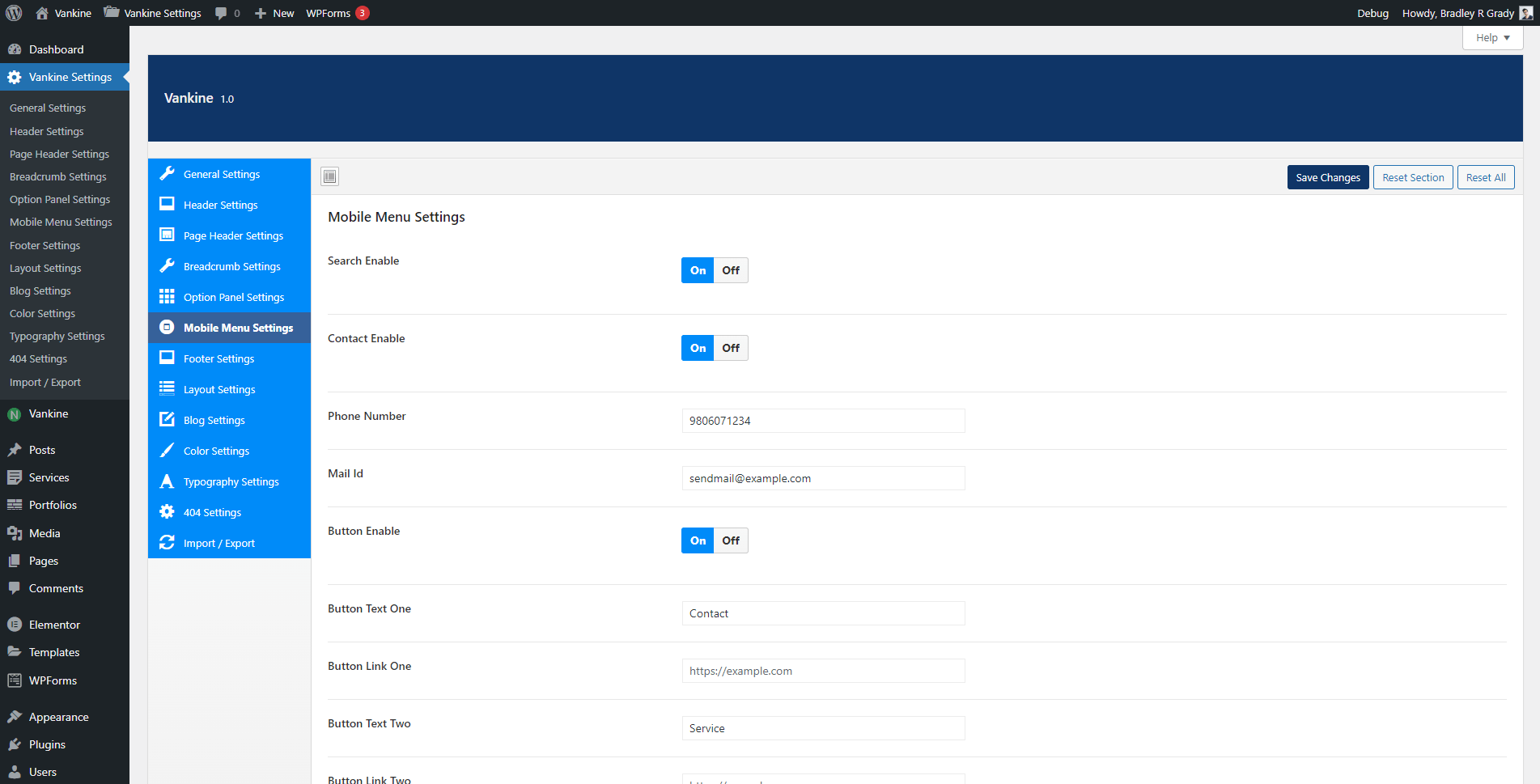The image is a screenshot of a computer interface for a website called "Vankin." At the top of the screen, there's a house icon followed by the name "Vankin." Below that, a folder labeled "Vankin settings" is visible. On the left side of the screen, there is a black vertical column with the word "Dashboard" at the top. Directly underneath, a blue bar highlights the current selection: "Vankin settings," indicated by a gear icon to the left.

The main section of the screen has a white background with a dark blue banner at the top left corner, displaying the word "Vankin." Below this banner, a blue vertical column lists various setting options. The "Mobile Menu Settings" option is highlighted about halfway down this list.

To the right of these menu options, the main content area details "Mobile Menu Settings." Several options are toggled on, including "Search Enable" and "Contact Enable." Below these toggles, there are fields for "Phone Number" and "Mail ID," with an input bar to the right for email information. 

Further down, another toggle labeled "Button Enable" is turned on. This section displays two sets of button configurations: "Button Text One" with a corresponding "Contact" field to the right, and "Button Link One" with a field to input a website address. Similarly, "Button Text Two" shows a box labeled "Service" to the right, followed by "Button Link Two" at the bottom, which again provides a field for a web link.

Overall, the screenshot captures a well-organized settings page for configuring the mobile menu options of the Vankin website.